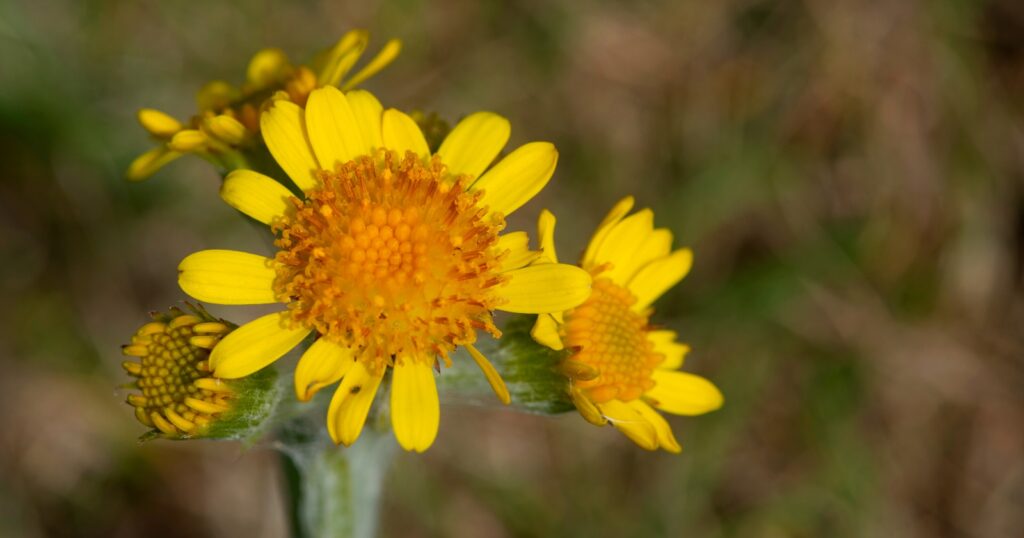This close-up image showcases a cluster of vibrant yellow flowers on a single green stem. The central flower, which is the largest and most clearly visible, is prominently in full bloom, revealing its intricate orange pollen and multi-layered, scalloped petals. Surrounding this main flower are several others: one to its right that is similarly open but not as large, another above facing the left corner, which is also fully bloomed, and a smaller bud lower down on the left, beginning to open. The background is blurred, presenting a mix of green, purplish, and red tones, implying a natural setting such as a garden or forest. Together, these blossoms create a striking visual with their layered petals and vivid yellow hues, framed against a mottled green and brown backdrop. The image captures the delicate beauty and varying stages of bloom within this cluster of flowers.